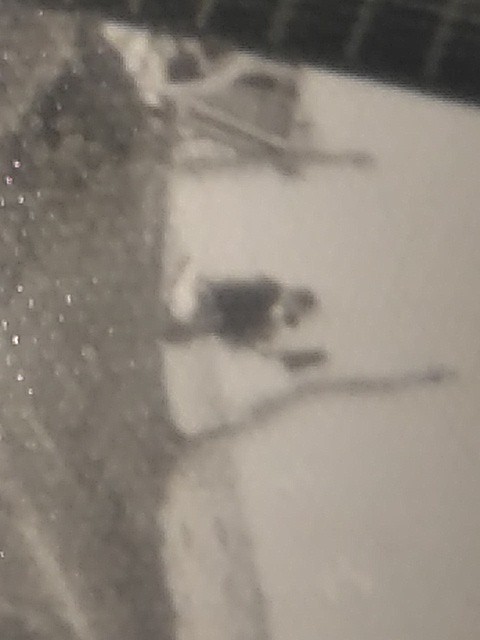The image showcases a black-and-white photograph, which appears slightly angled and disorientingly blurry, as if viewed through a textured film like bubble wrap or a similar sheer plastic covering. The photograph itself appears to document an older, gray-tone photograph, compounding the blur and obscuring details. A man dressed in a black jacket and gray pants can be seen sitting and holding an unidentified object in his hands. Beside him is a light gray vehicle with darker gray accents, though specifics are difficult to discern due to the fuzziness. The composition is portrait-oriented but could be intended to be horizontal, contributing to the distorted perception. The top fifth of the image includes a dark gray to black background, while the right side is predominantly white with some black, indiscernible objects. The bottom shows a mix of dark gray that fans out diagonally, alongside areas of light gray to white. The background features a wall with dark gray bricks and white grounding elements. This complex layering and texture give the image a surreal, almost snakeskin-like appearance.